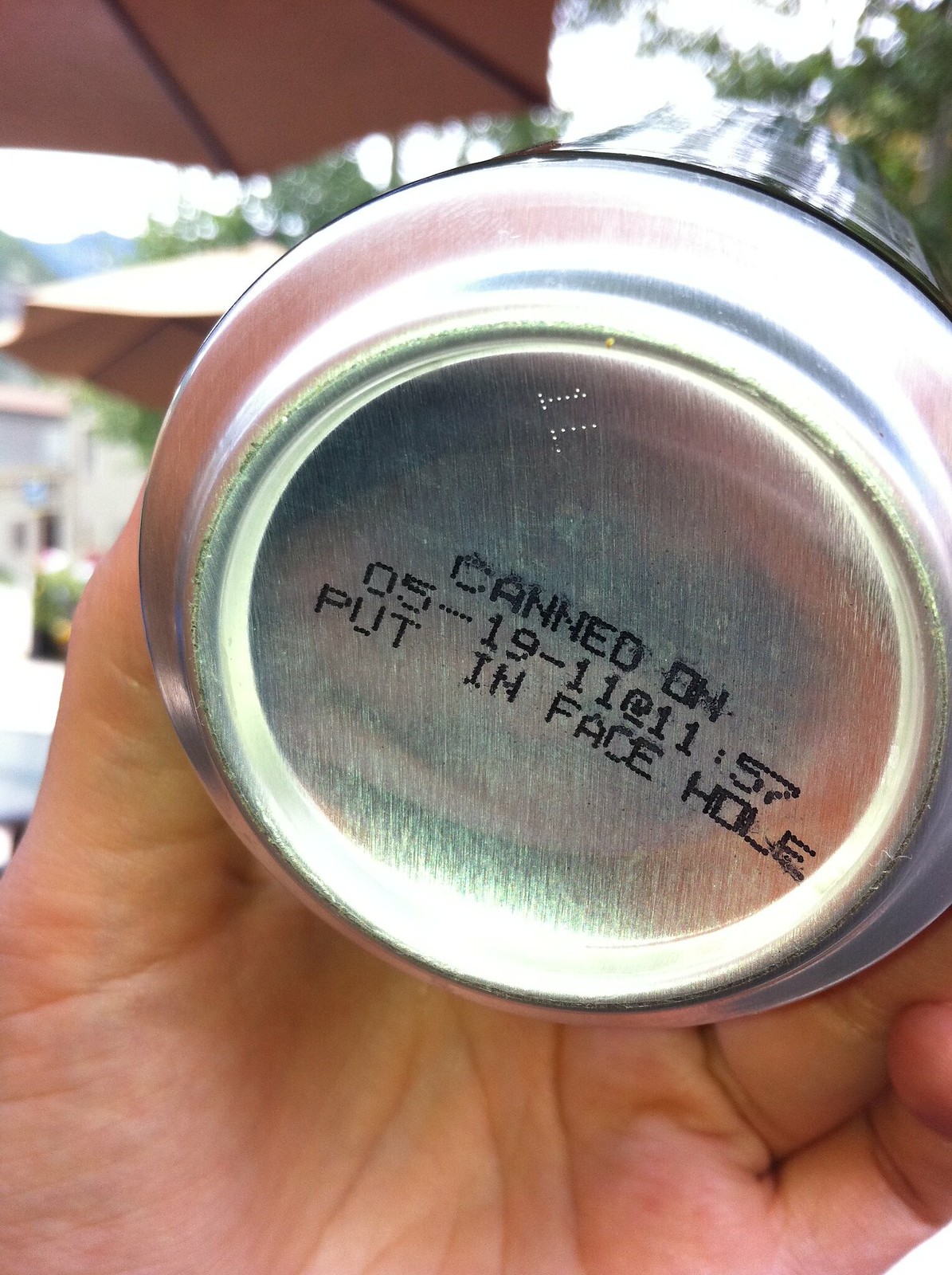This close-up photograph captures a white left hand holding the bottom of a soda can, showcasing its silvery metal base. The bottom of the can displays black text reading "canned on 05-19-11 @ 11:57" followed by "put in face hole." The perspective reveals the hand cupping the can, emphasizing the silver bottom. Reflections of light and tree leaves are visible on the can, with blurry leaves appearing in the upper right of the image. The background includes a dark red umbrella at the upper left, patches of sky, and more tree leaves, adding depth to the composition.